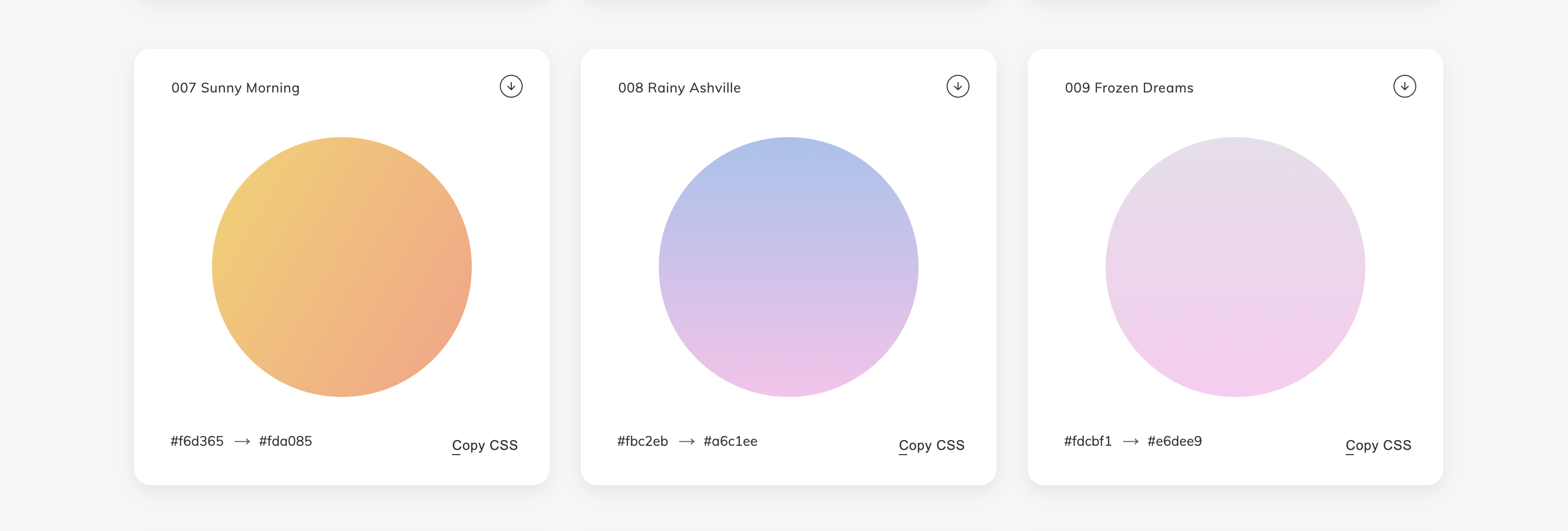The image features a rectangular box with a light purplish-gray color. Inside this box, there are three white squares, each containing detailed information:

1. The first square (on the left) displays the text "007 Sunny Morning" at the top. Below this text, there's a downward-pointing arrow encased in a circle. The center features a large orange circle. At the bottom, it provides the hexadecimal color code "#F6D365" along with a sideways arrow pointing right. Next to this, the text reads "Copy CSS" and the CSS color code "#FDA085".

2. The middle square is labeled "008 Rainy Asheville" at the top. A circle containing a downward-pointing arrow is located below this text. The main graphic element is a large circle, which transitions from a blue color at the top to a light purple at the bottom. The bottom area features the hexadecimal color code "#FBC2EB" with a right-pointing arrow beside it. It also includes the text "Copy CSS" next to the CSS color code "#86C1EE".

3. The third square (on the right) begins with the text "009 Frozen Dreams" at the top. The description for this square ends here, suggesting that additional details might be present but are not included in the provided transcript.